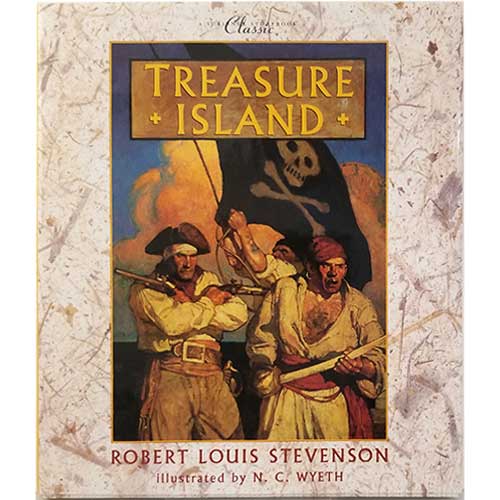This illustrated cover for "Treasure Island" by Robert Louis Stevenson, featuring artwork by N.C. Wyeth, is part of a classic book series and depicts a highly detailed and atmospheric scene. Three pirates, clad in traditional pirate attire, dominate the cover. The central pirate on the left brandishes two revolvers with a determined expression; he wears a captain's hat, a white collared shirt unbuttoned down the chest, a belt, a sash, and gray pants. The rightmost pirate grips a scimitar eagerly, adorned in a red headscarf, an open white shirt revealing his chest, a red sash, and white pants. In the background, a third pirate hoists a black pirate flag emblazoned with a skull and crossbones, his arms outstretched toward the moody sky. The scene is imbued with dark, brooding colors, including moody blues and pinks that suggest a stormy backdrop. The title "Treasure Island" is prominently displayed in yellow on a wooden plank at the center, framed by a neutral cream-colored, stone-like outer border that adds a classic touch to the cover's composition.